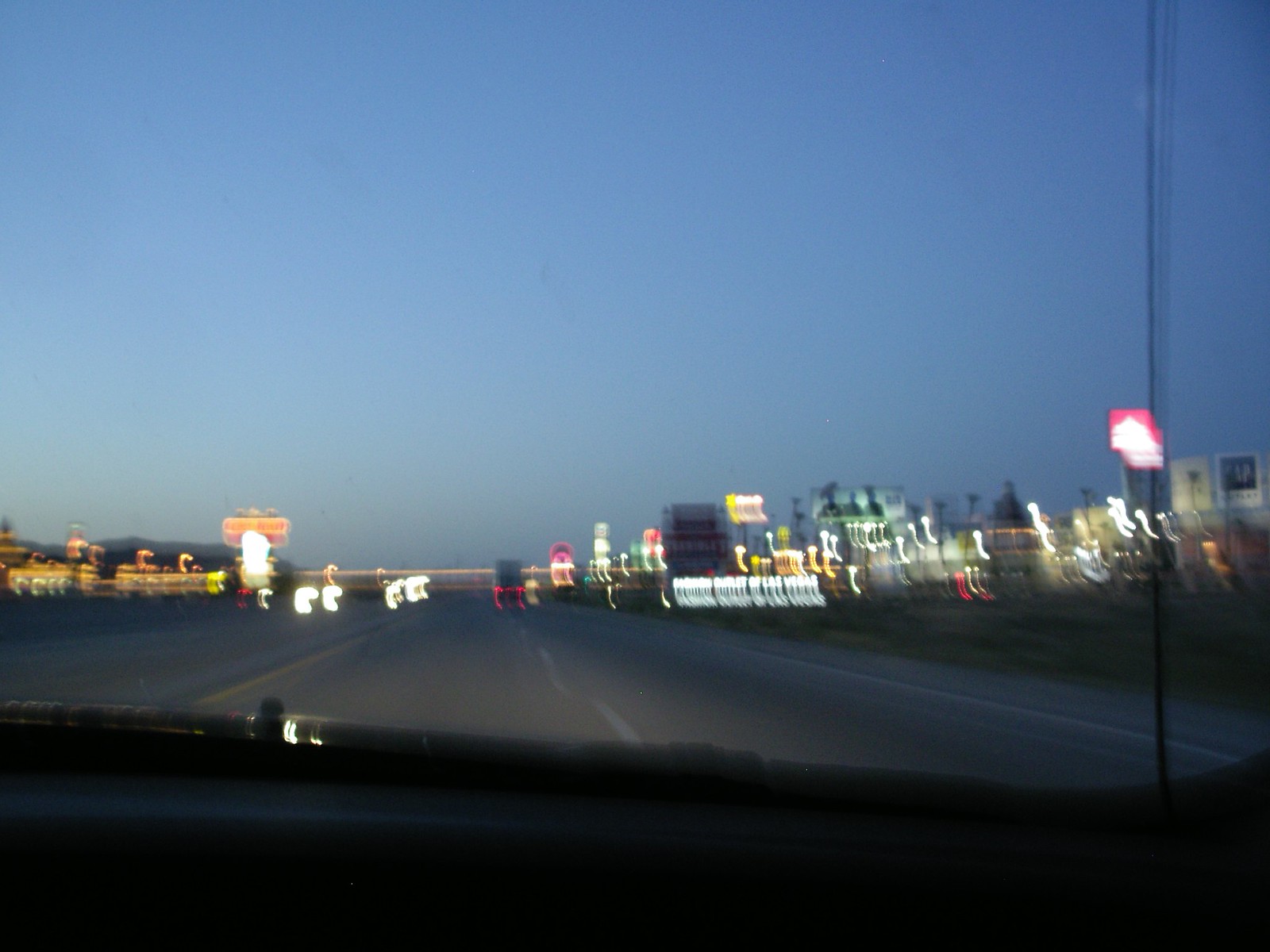The photograph, although very blurry, captures a freeway scene approaching nighttime, likely set in the western United States. It appears to be taken from inside a vehicle, through a windshield, depicting a busy roadway with big rig trucks and other cars. The freeway lacks a center divide and features a left-turn lane. The horizon is dotted with hotels and food joints, their lights beginning to illuminate the cityscape. The background reveals a city with its colorful, blurry lights, giving it the appearance of a hazy, luminous blur. Water is visible in the distance, reflecting the ambient city lights. The sky transitions from a darker blue to a lighter blue towards the left, indicative of the sun setting or partially set. There's a prominent red sign at the top right of the image, contributing to the modern yet slightly overwhelming visual clutter. The overall scene exudes a mix of urban and twilight ambiance, despite the photograph's poor clarity.